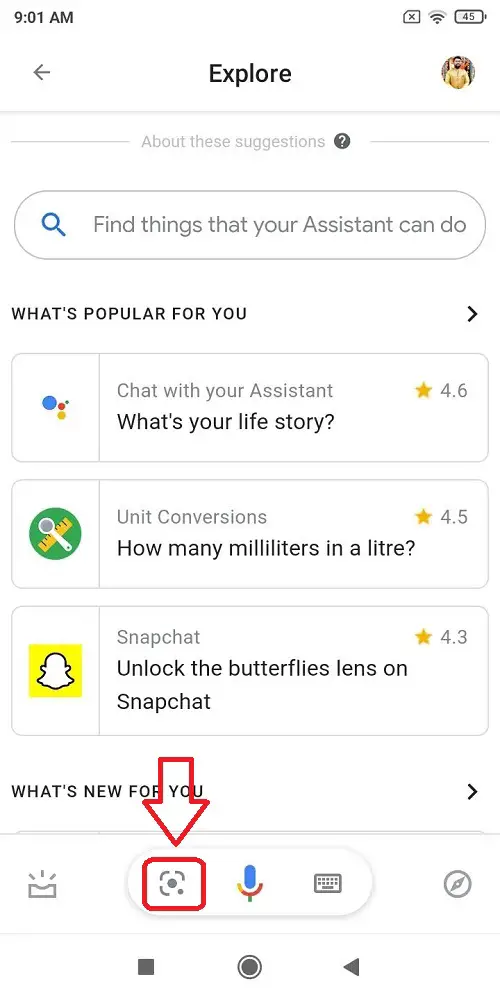This image is a screenshot taken from a smartphone, displayed vertically within the upper left-hand corner of the page. The device's status bar at 9:01 a.m. shows a Wi-Fi indicator and a battery status at 45%. 

Centered at the top of the screen, the text "Explore" is visible along with a small, barely discernible profile picture on the far right, likely depicting a male in a yellow shirt. Below this, the screen features the phrase "About these suggestions" followed by a prominent search bar that reads "Find things that your assistant can do."

Further down, under the section titled "What's popular for you," there are several content suggestions including "Chat with your assistant," "What's your life story," "Unit conversions: How many milliliters in a liter?", and "Snapchat: Unlock the butterflies lens on Snapchat."

An eye-catching large red outlined arrow is placed over the text "What's new for you," pointing downward towards a camera icon, which itself is highlighted by a red square outline.